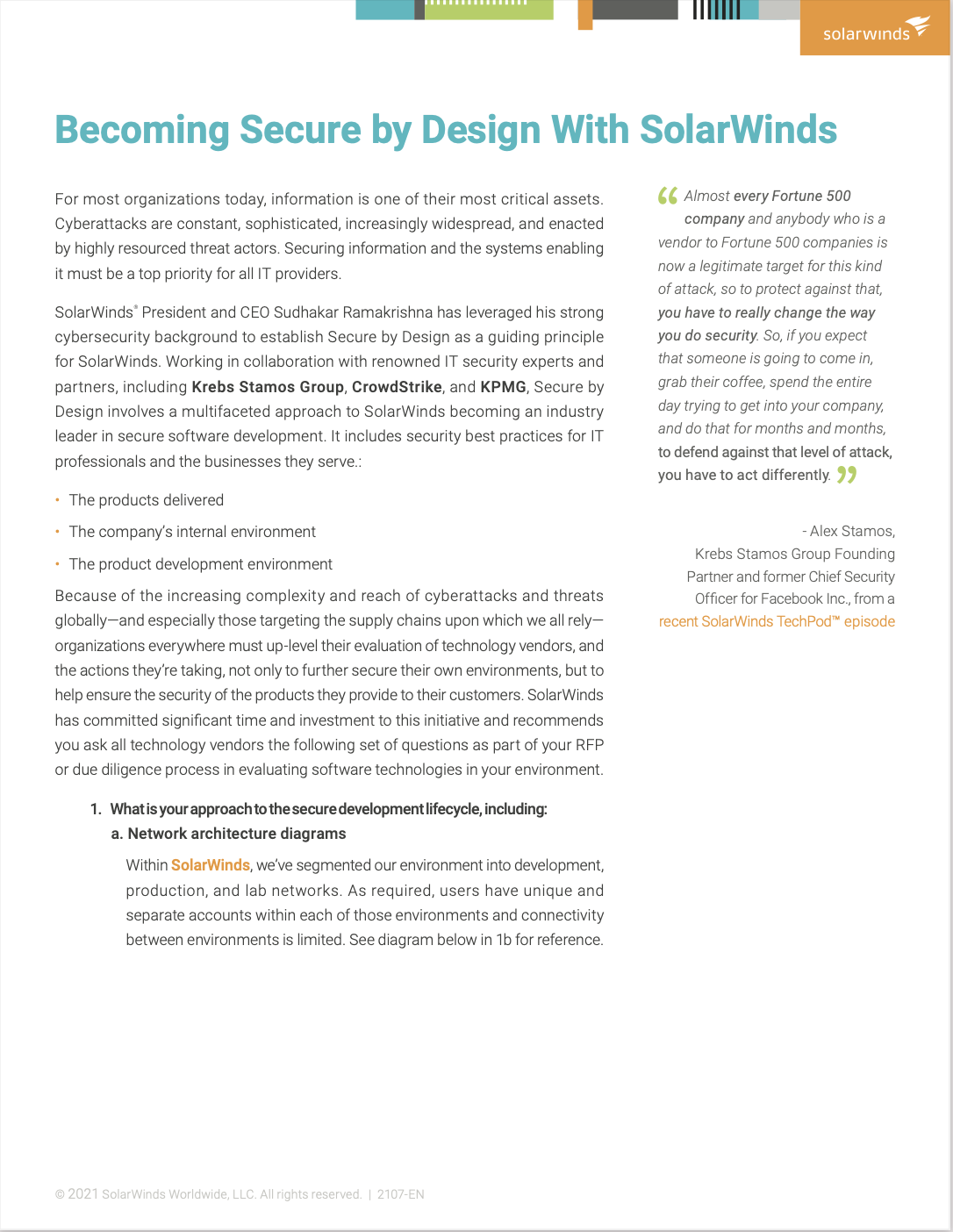The image resembles a textbook page, distinctly labeled with "SolarWinds" in the upper right corner. The heading reads, "Becoming Secure by Design with SolarWinds." It emphasizes the importance of information security in today's organizations, highlighting that cyberattacks are relentless, sophisticated, and perpetrated by highly skilled adversaries. Consequently, safeguarding information and the systems that manage it is imperative for all IT providers.

Sudhukur Ramasheema, SolarWinds' President and CEO, has utilized his extensive background in cybersecurity to make secure design the company’s foundational principle. He collaborates with esteemed IT security experts and partners, including Krebs, the Stamos Group, CrowdStrike, and KPMG.

The concept of "Secure by Design" at SolarWinds entails adopting a comprehensive strategy to lead the industry in secure software development. This approach integrates security best practices essential for IT professionals and the businesses they support. The company's commitment extends to reinforcing both its internal and product development environments.

Given the escalating complexity and prevalence of cyberattacks, specifically targeting global supply chains, organizations are urged to elevate their scrutiny of technology vendors. This involves not only ensuring the security of their own infrastructures but also confirming the security commitments of their vendors' products.

SolarWinds has dedicated significant resources and investment to this initiative. They advise organizations to include a specific set of questions in their Request for Proposal (RFP) or due diligence process when assessing software technologies to ensure thorough evaluation and enhanced security.